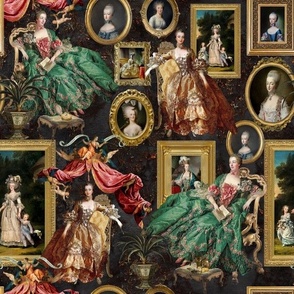A visually engaging artwork features a collage of numerous framed portraits against a black textured wall, depicting women from what appears to be the Victorian or Marie Antoinette era. The top left corner hosts a striking portrait of a woman in a green and red dress, seated in a black chair, holding a book in her left hand, faced rightward. Adjacent to her is a pot with a green plant. Artfully arranged around this central figure are a myriad of frames, including several gold-bordered ones. Noteworthy are two oval portraits of women facing opposite directions, followed by another gold-framed, indiscernible square picture, and more portraits of women, often adorned in opulent attire.

Further right, a woman in a long, flowing brown dress sits elegantly, facing the camera. Behind her, a mother and her two children are captured in a gold-framed square portrait. The top right corner is adorned with another gold-framed image of a woman, below which lies an oval-shaped picture of a woman, and further down, a circular portrait. In the foreground, another woman in a green dress with a red front sits, holding a book across her lap, facing the viewer.

Centrally, a partial view of a gold-bordered portrait reveals a woman. To the right of this, an unclear image resembles a big red gown. Additionally, below these elements is a woman in a brown dress, seated like the one in the top right, beside a larger version of the portrait featuring the woman and two children. The walls capture elements of French Baroque style and are interspersed with drawings of women lounging in luxurious chairs, accentuating their grandeur and elegance. The presence of plants in the background adds to the textured intricacy of this elaborate visual ensemble.